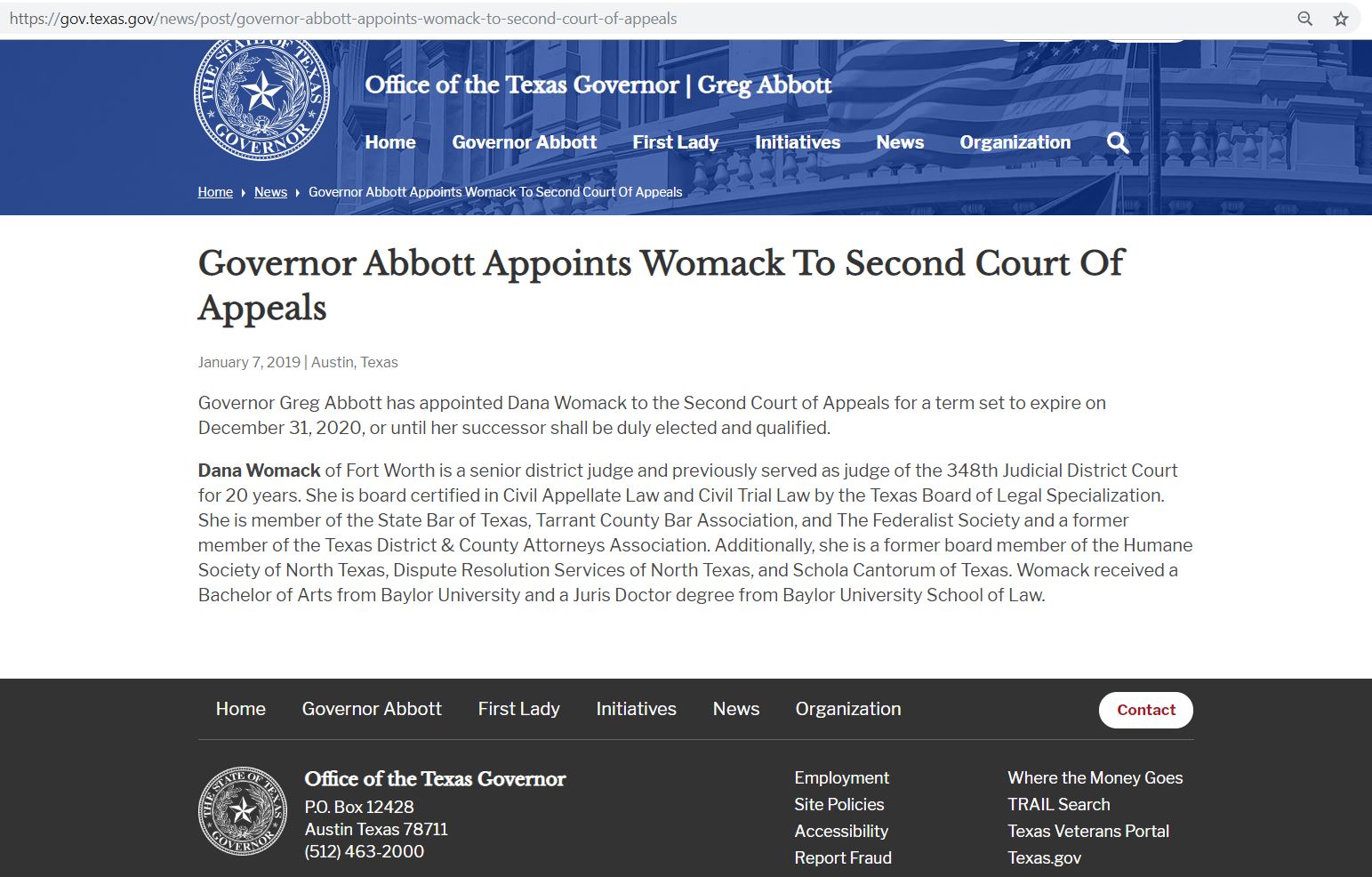The image is a screenshot of the Texas Governor's official website. At the upper left-hand corner, the web address 'gov.texas.gov' is prominently displayed. Below the web address is a horizontal blue bar stretching from left to right, adorned with a close-up image of a government building with a flag proudly flying above it. In the foreground, the text 'Office of the Texas Governor' is clearly visible, accompanied by the name 'Greg Abbott'.

Beneath this section is a navigation banner with the following labels: 'Home,' 'Governor Abbott,' 'First Lady,' 'Initiatives,' 'News,' and 'Organization.' Additionally, a magnifying glass icon indicates the search function.

At the bottom of the banner, there's a headline that reads: 'Governor Abbott appoints Womack to Second Court of Appeals,' and it's dated January 7, 2019.